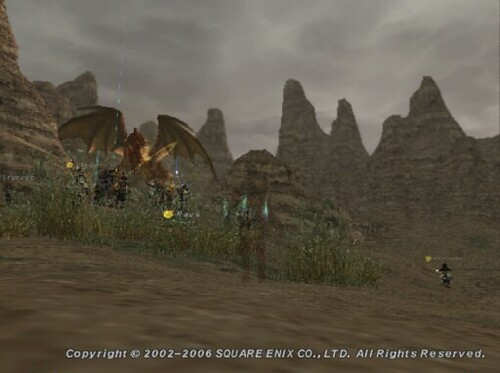This digital artwork, set within a rectangular frame, features a dynamic and surreal mountainous landscape under a dark gray, streaked sky. Dominated by gray and dark gray rocky formations, some with gold and yellow streaks, the terrain showcases pointed, pyramid-like peaks that create a rugged mountain terrain. Towards the lower section of the image, patches of greenery and various shades of brown sand - possibly dirt or a dirt path - contribute to an uneven foreground.

Superimposed over this terrain are various futuristic figures, including a creature reminiscent of a flying pterodactyl or dragon in the left center, adorned with golden highlights. Additionally, there are other fantastical creatures positioned amidst the scene; one stands prominently in the sandy foreground while another is situated to the right. These figures are illuminated by blue and yellow lights, enhancing their otherworldly presence against the natural backdrop.

At the base of the image, a white text copyright notice reads, "Copyright 2002 to 2006, Square Enix Company Limited, all rights reserved," indicating the timeframe and ownership of this striking digital composition.